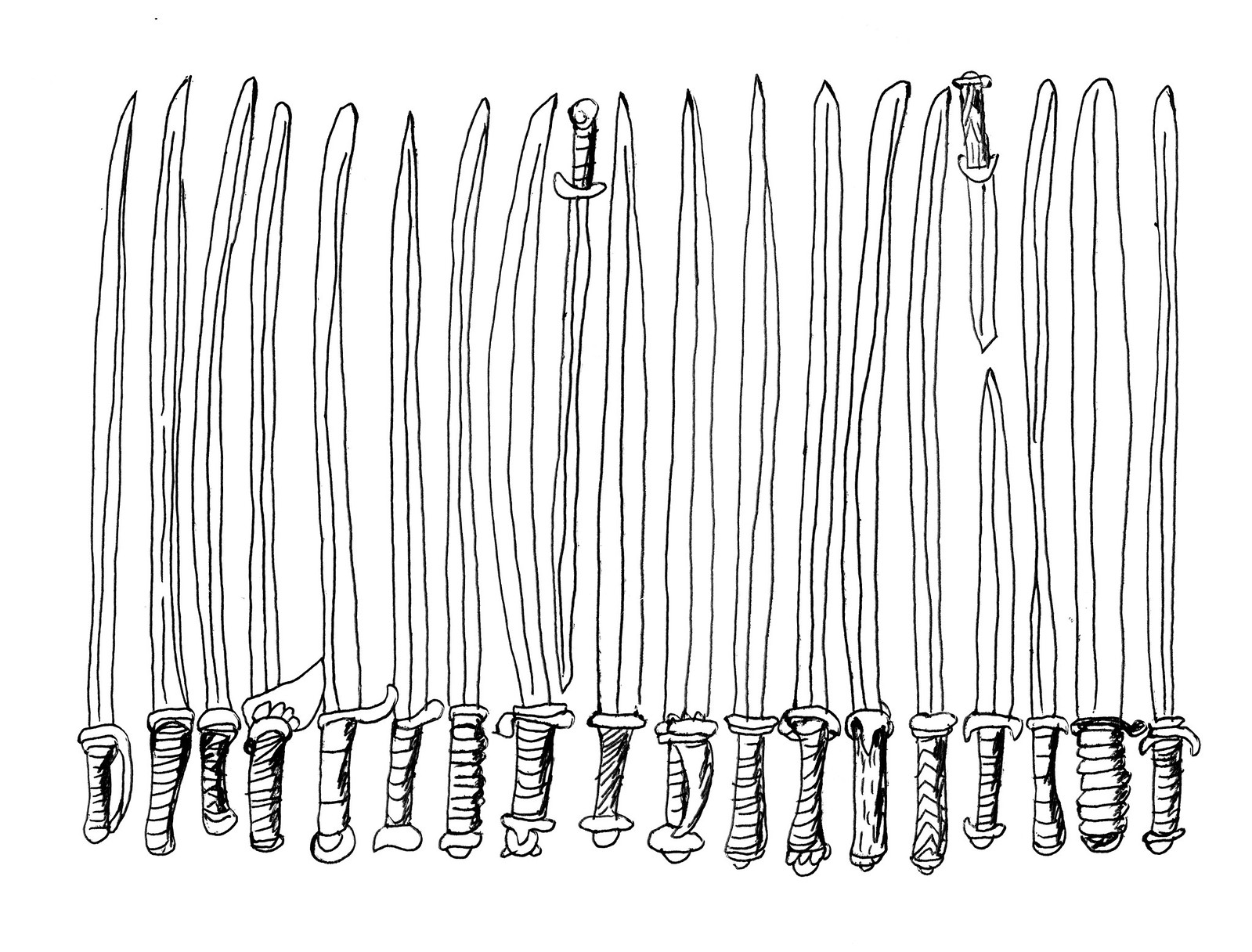This image is a black-and-white line drawing showcasing approximately 15 to 20 swords, all displayed vertically against a plain white background. The swords, predominantly long and medieval in style, are positioned with their hilts at the bottom and blades pointing upward, except for two shorter swords—or possibly daggers—with handles at the top and blades pointing downward. The illustration is rendered in very sketchy black ink, characterized by wobbly, uneven, and non-straight lines, giving the artwork a crude yet appealing appearance. The hilts of the swords exhibit different designs with varied guards and handles, shaded with black scribbles to differentiate each one. Despite the simplicity and wonkiness of the line art, the repetitive arrangement of the swords creates a visually engaging pattern.